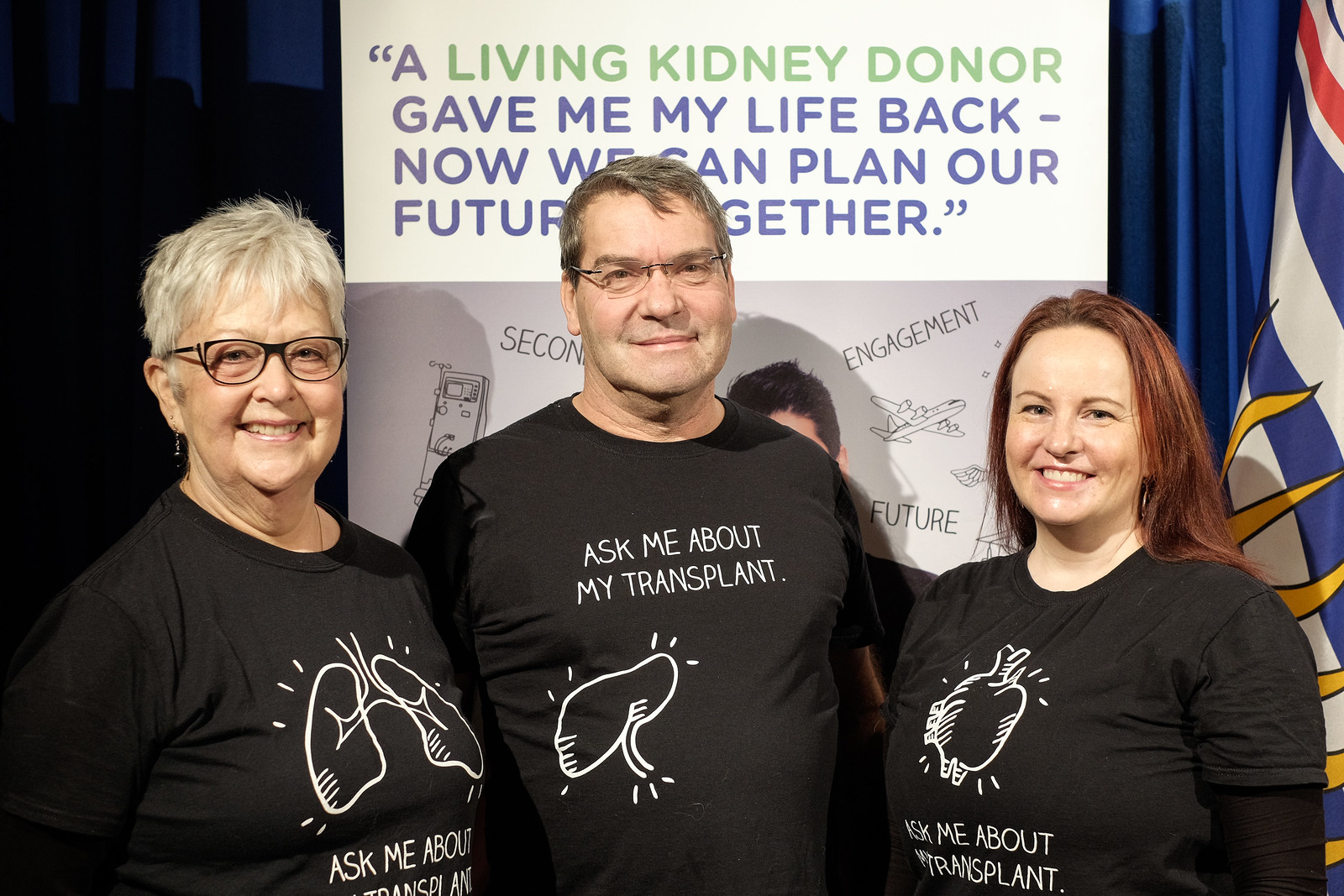In this indoor setting, the photograph captures three individuals standing side by side at the center of the frame, directly facing the camera and smiling. The trio consists of two females, one with very short gray hair on the left and another with long red hair on the right, and a male with glasses positioned between them. All three are dressed in matching black t-shirts with white letters reading "Ask me about my transplant," each featuring a different organ illustration: lungs on the gray-haired woman’s shirt, a kidney on the man’s shirt, and a heart on the red-haired woman's shirt.

Behind the group is a prominently displayed white sign with green and blue lettering, stating: "A living kidney donor gave me my life back. Now we can plan our future together." Below this text are partially visible drawings and words, including "engagement," "future," and an image of an airplane and what might be a cellphone. The background is adorned with bright blue curtains on either side and a state flag on the right, suggesting the photo was taken on a stage during a charitable event. The vivid colors in the image—including red, white, blue, green, black, gray, yellow, and orange—add to the lively and hopeful atmosphere depicted in this powerful moment of advocacy and gratitude.